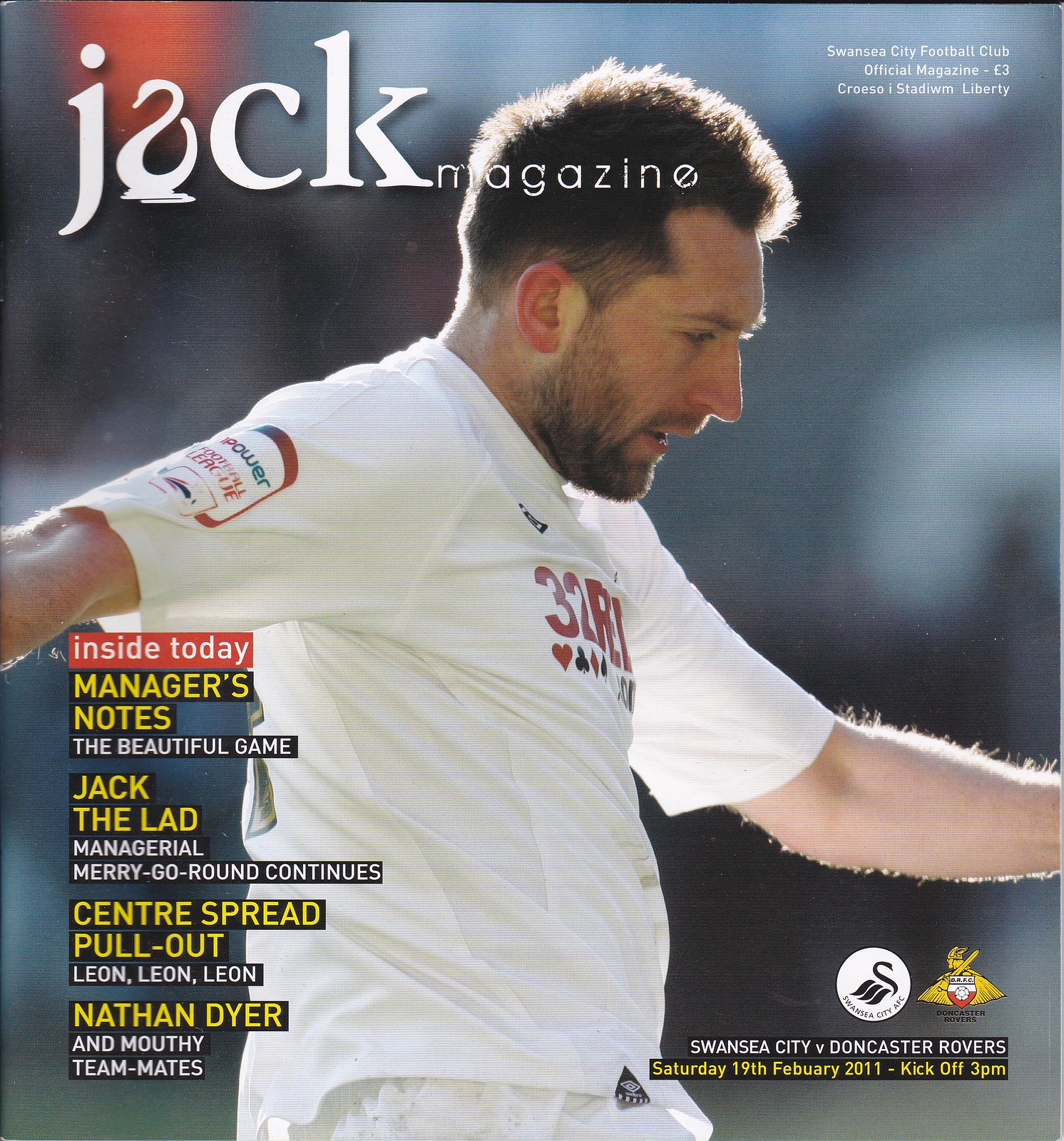The magazine cover is titled "Jack Magazine," though the second letter 'a' is stylized as a swan, creating some ambiguity. This official magazine of Swansea City Football Club is priced at three British pounds. The cover features a soccer player in a white uniform with red lettering and white shorts. The player has a beard and whitish hair, and he is depicted in motion with his right arm extended to the left and his left arm down to the right, possibly in the act of kicking a ball. The background is blue, indicating an outdoor setting. 

Text on the left side of the cover includes yellow and white print listing the contents: "Inside Today," "Manager's Notes," "The Beautiful Game," "Jack the Lad," "Managerial Merry-Go-Round Continues," "Center Spread Pullout," "Leon, Leon, Leon," "Nathan Dyer," and "Mouthy Teammates." The bottom right corner displays logos of Swansea City and Doncaster Rovers, with match details: "Swansea City versus Doncaster Rovers, Saturday 19th February 2011, kickoff 3 p.m."